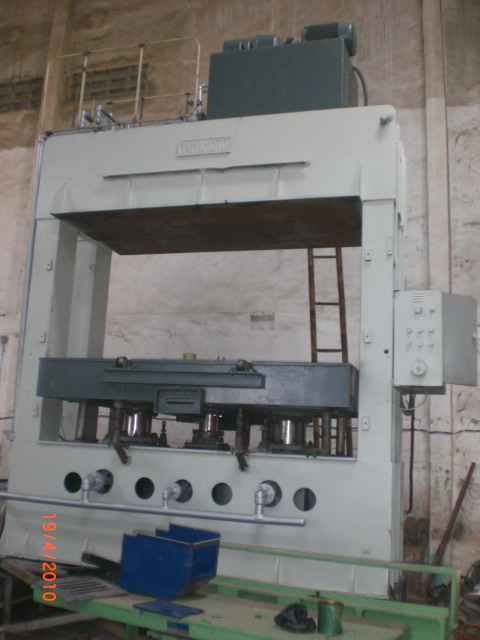This color photograph, taken in portrait orientation, captures the interior of a high-walled factory facility or machine shop characterized by walls that are light cream at the bottom and dark gray towards the top. The focal point of the image is a vertically-oriented mechanical instrument, likely a drill press or machine press, situated against the wall. This machine features a substantial gray, oblong rectangular box at its center, with a silver pipe protruding from below. Above this central box is a ladder leading to a ledge that supports a shorter, but taller, gray rectangle. Below the central box, there are metal projections or silver cylinders extending downward. 

The front of the machine is equipped with a row of control buttons and knobs, three of which have silver turn handles connected to a large vertical bar. In the foreground, there is a table or cart with light green metal sides and a blue object resting on its top left corner. Additionally, a large gray structure resembling a power unit is positioned at the top of the machine. The overall style of the photograph is representational realism, capturing the intricate details and industrial atmosphere of the machine and its surroundings.